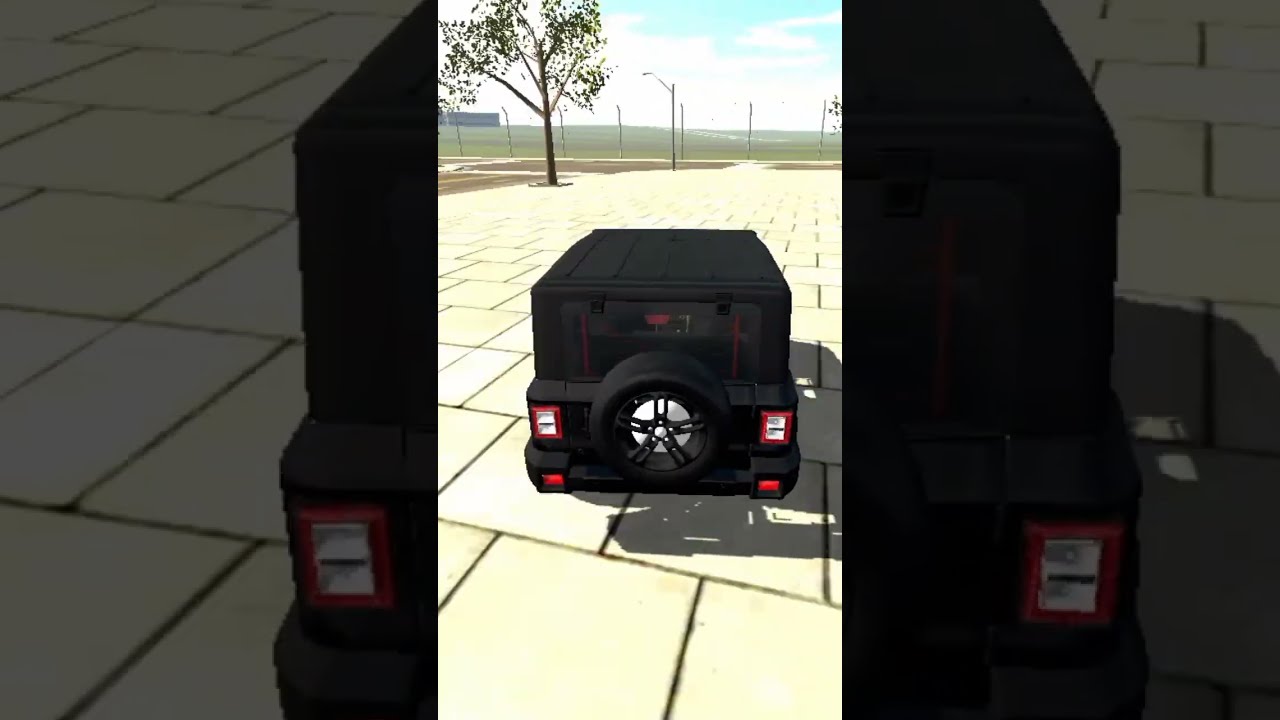The image captures a detailed, possibly simulated scene reminiscent of a video game. At the center is the back end of a sturdy, black Jeep or SUV, distinguished by its large black wheel with black spokes mounted on the rear. The vehicle’s taillights have a striking red outline with white rectangles embedded within them. It’s parked on a surface of large, cream-colored brick tiles, resembling the kind of pavement you might find in a park.

This photograph-within-a-photograph composition features a shaded overlay on the left and right thirds, highlighting the central part of the image. The entire background, a blown-up and darkened version of the SUV itself, creates a frame around the main subject.

In the upper left-hand corner, there is a thin-trunked tree with a few green leaves. Extending further into the distance, the scene reveals a green field with brown patches, dotted with gray street light poles and large metal fence posts. The sky above is a vivid blue, dappled with white, puffy clouds, indicating a bright daytime setting. All these elements are captured from a slightly elevated, top-down angle that allows for an expansive view of both the SUV and its surroundings.